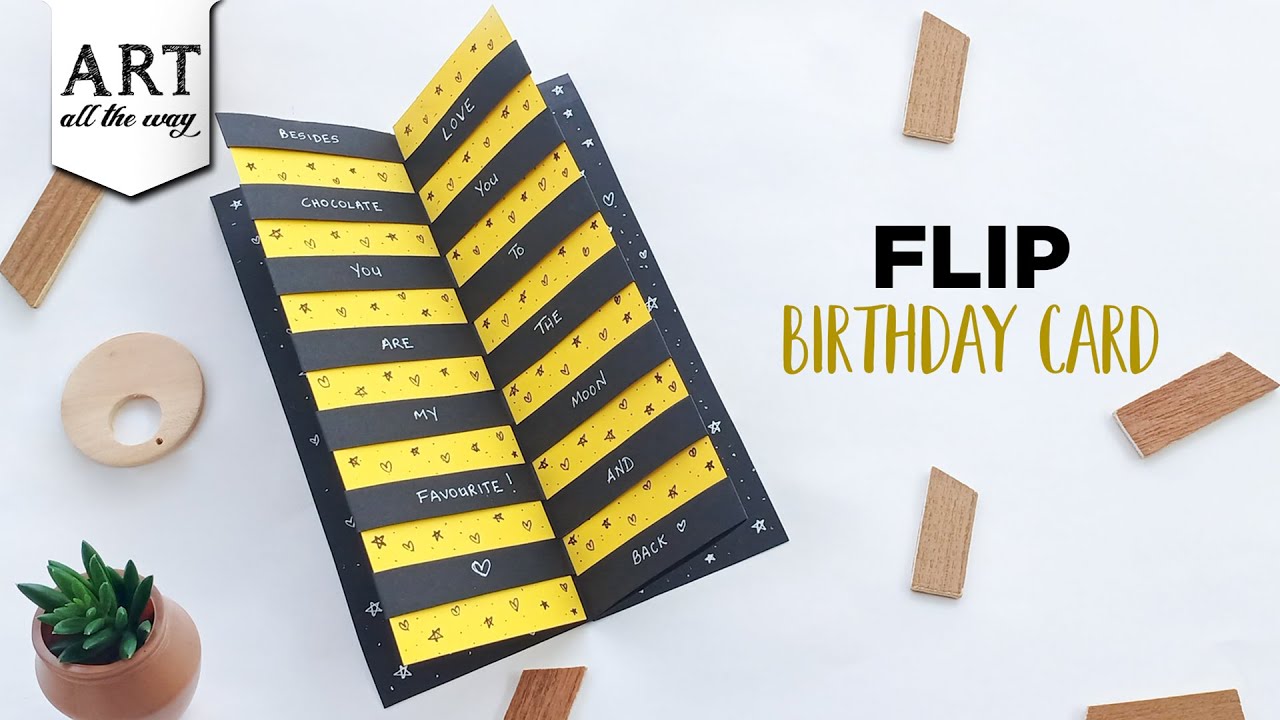This image depicts an indoor arts and crafts project, likely a how-to tutorial for creating a "Flip Birthday Card." Dominating the image is a two-toned, black and yellow card, expertly crafted from paper. Located on the top left is a white banner with the words "Art All the Way" in black text. The card itself is intricately designed with multiple strips that flip to reveal hidden messages. On the left side, a black strip reads "besides," followed by a yellow strip adorned with hearts, another black strip with the word "chocolate," and a final yellow strip that says "you." The card is surrounded by various items including wood pieces, a small plant in a pot on the bottom left, and a round wooden piece on the right. The right side of the image features black text reading "flip," and directly below it, in yellow, the text "birthday card." The overall atmosphere is that of a step-by-step guide, demonstrating how to assemble this creative and heartfelt birthday card.